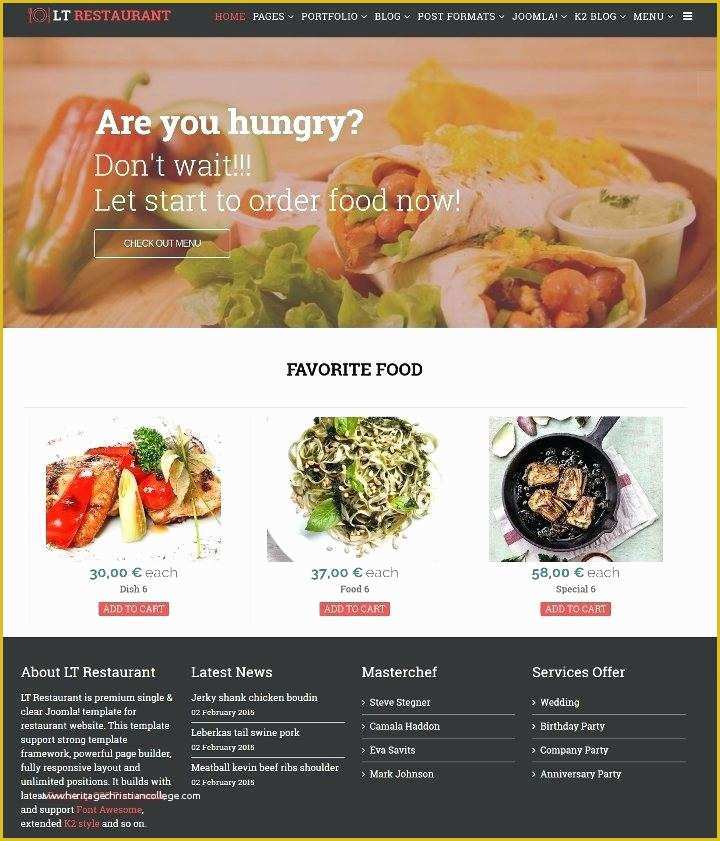The image is a screenshot of a restaurant's menu. In the top left corner, there is a heading that reads "LT Restaurant." To the right of this heading, several page sections or categories are listed, including "Home Pages," "Portfolio," "Blog Post Formats," "Joomla!," "K2 Blog," and "Menu."

The main portion of the page features a message inviting customers to order: "Are you hungry? Don't wait! Let's start to order food now." Below this message, there is a clearly marked button labeled "Checkout Menu."

Further down, the menu highlights some favorite foods, listing three different dishes. The first dish is labeled "Dish Six" with a price of €30. The second is "Food Six" priced at €37, and the third is "Special Six" with a price of €58. The currency appears to be in euros (€).